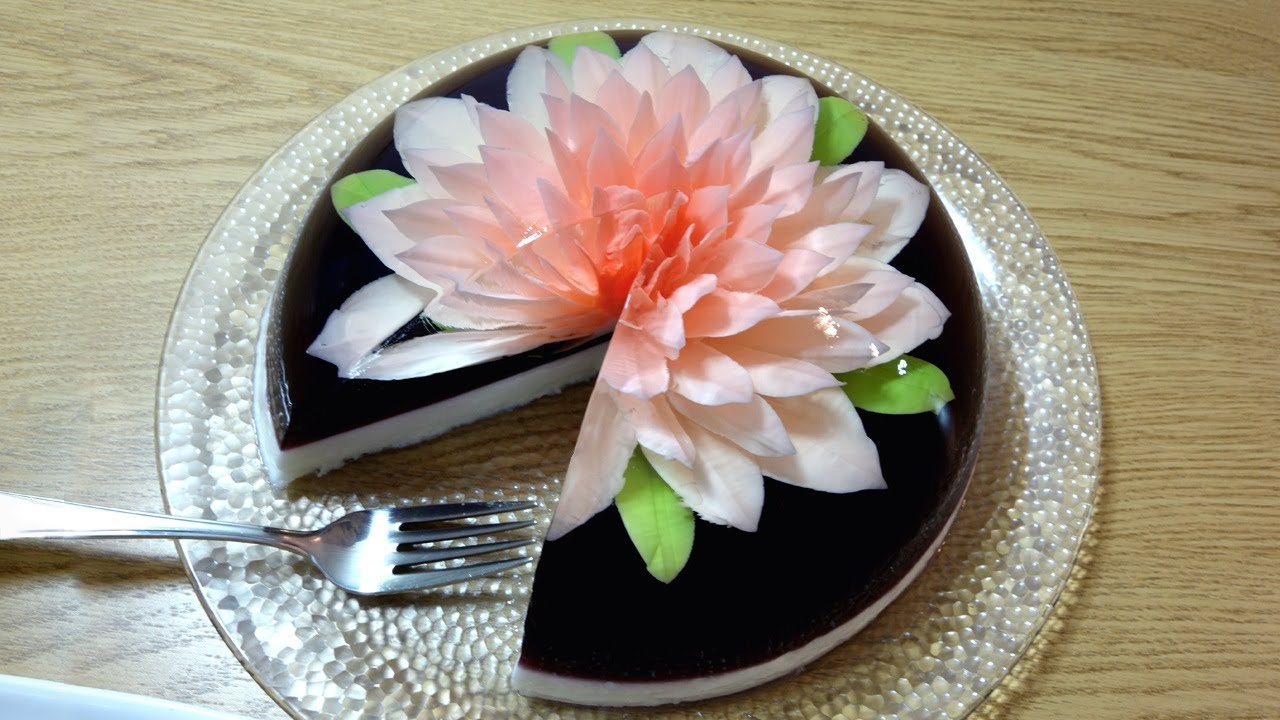This horizontal rectangular image displays an elegantly presented cake that has been cut to reveal its multi-layered structure. The cake itself, round and resembling the size of a standard cake pan, features a dark brown, possibly chocolate top layer. A slice has been taken out, revealing a pristine white filling beneath the dark top layer. The base of the cake appears to have a graham cracker crust or a similar type of crust, although this detail is somewhat ambiguous.

The cake is meticulously placed on a circular, iridescent platter with white dots, which adds to its visual appeal. Above the cake, there is a stunning pink flower that spans almost to the cake's edge, with delicate petals in shades of pink and white. This flower decoration maintains its form even after a wedge of the cake, part of the flower included, has been removed.

Resting to the left on the fancy, see-through plate is a clean silver fork, ready for the next person to enjoy a piece. The entire setup sits atop a tan, wooden table with a distinct grain pattern, enhancing the overall rustic yet sophisticated presentation of the dessert.